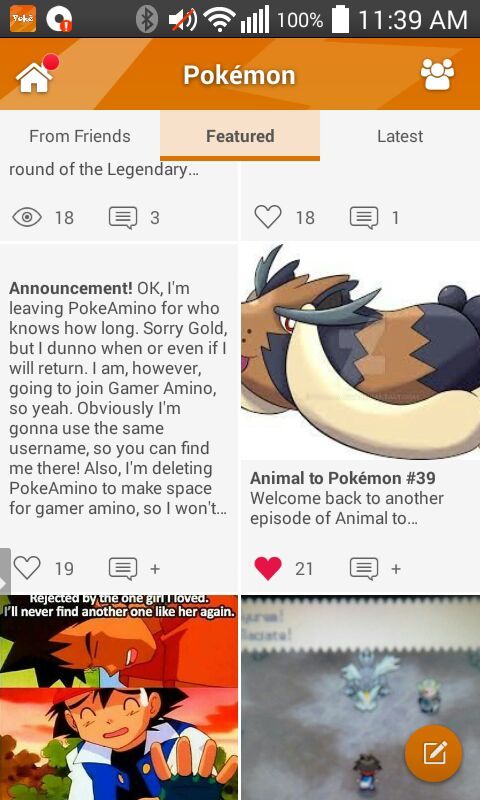This descriptive caption details a screenshot from a mobile device, potentially a phone or tablet. In the upper left corner, there's a grey notification bar. Within this bar, there's an orange square with rounded edges showcasing a gradient effect, featuring what appears to be four letters spelling "Pokey." Adjacent to it, there’s a circle bordered by a thick white line and a smaller red circle within it at the bottom right, displaying a white exclamation mark. Also visible are a Wi-Fi signal icon, a muted sound icon denoted by a red stripe, a battery indicator at 100%, and the time indicating 11:39 AM.

Just below this, there is an orange gradient tab. On the left side of this tab, a white icon depicting a house with a red circle atop the chimney is present, and centrally, the word "Pokemon" is displayed in white font. To the right side, a white icon representing a group of people is visible. Below, there are three tabs labeled "From Friends," "Featured" (which is selected and highlighted in light orange), and "Latest."

The next section reads "Round of the Legendary..." followed by an eye icon with the number 18 and a comment icon with the number 3. The subtitle "Announcement" introduces a message: "Ok, I'm leaving Pokemon Poke Amino for who knows how long. Sorry Gold, I don't know when or even if I will return. I am however going to join Gamer Amino. So yeah, obviously I'm going to use the same username so you can find me there. Also, I'm deleting Poke Amino to make space for Gamer Amino. So I won't..."

The subsequent post features an image of a brown and grey Pokemon with long white ears, liked 18 times with one comment. It is captioned "Animal 2 Pokemon, number 39. Welcome back to another episode of Animal 2..." Further down, another image is liked 19 times with no comments, showing two main characters from Pokemon and a caption: "Rejected by the one girl I loved, I'll never find another one like her again." The final item, liked 21 times with no comments, appears to be an aerial view presumed to be from a Pokemon game.